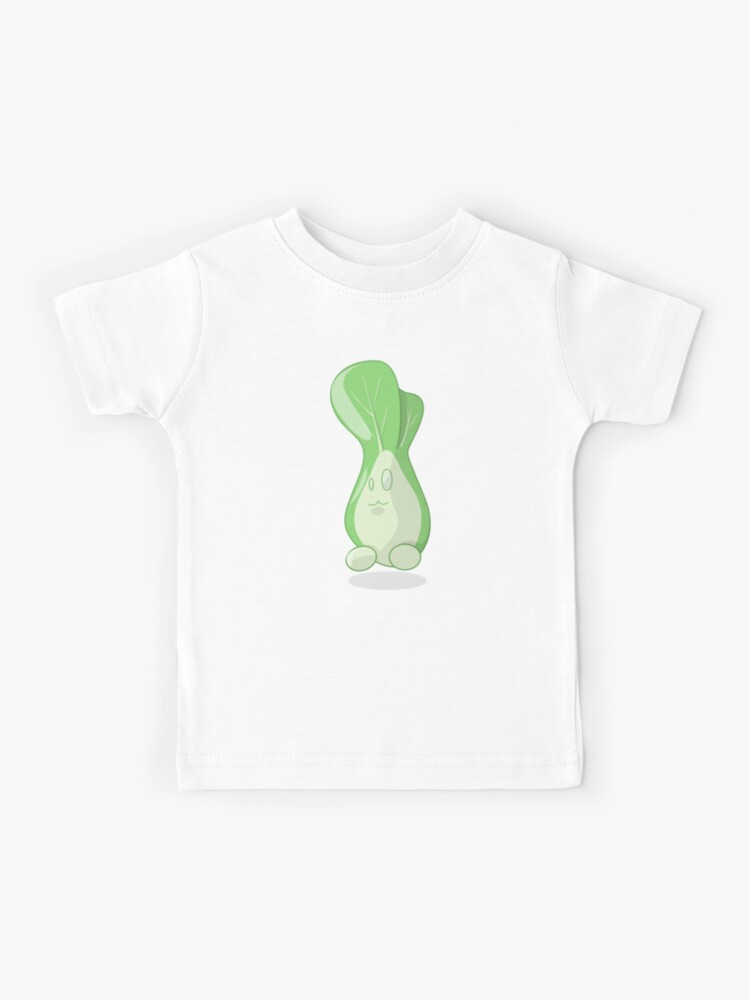In the image, a simple white scoop neck T-shirt is displayed against a plain white background. The T-shirt features an intriguing design at its center. The design depicts two heads of lettuce, with the larger leaf positioned in front and the smaller one slightly behind it. The lettuce leaves are a soft, light green color. The central figure appears as a whimsical, anthropomorphic lettuce character with a body shape reminiscent of a potato or avocado but in a creamy hue, lighter than the T-shirt itself. This figure has one small green eye, a larger eye, a small mustache-like detail, and a tiny mouth, all accentuating its face. Two small round shapes at the bottom serve as feet, completing the quirky character. A delicate shadow beneath the figure adds depth and dimension to the playful design.